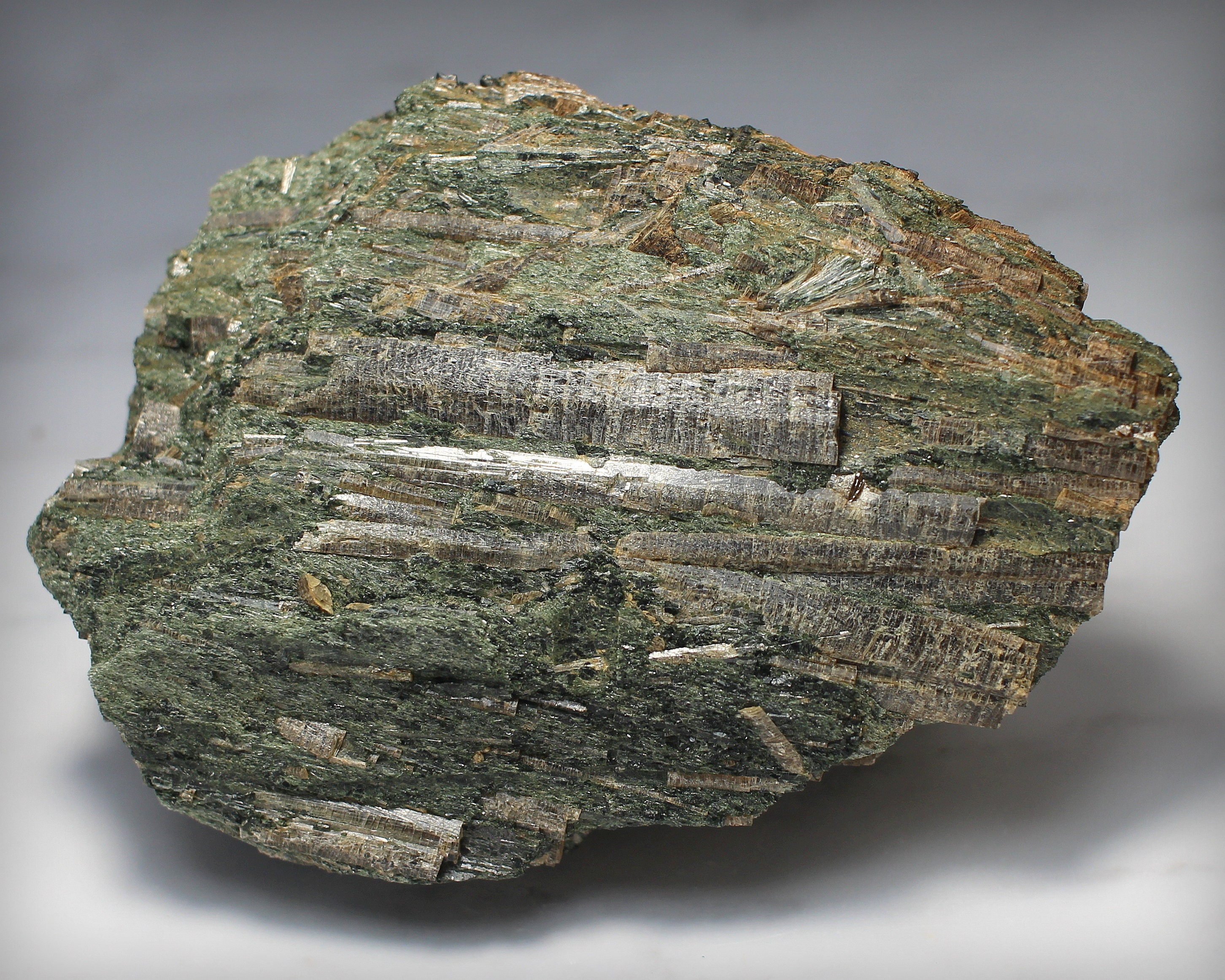The image depicts a large, oblong rock or mineral formation displayed on a light gray, seemingly museum-like background. The rock, possessing an irregular shape, showcases a blend of greens, grays, and browns, with notable lighter green hues on top and darker shades of gray towards the bottom. Additionally, brown rust-like coloration can be observed along the right side. Its surface features intricate etched lines running horizontally and vertically, offering a fossil-like or possibly petrified wood appearance. The rock is illuminated dramatically, casting a soft shadow with a faint white halo, enhancing its detailed and textured facade, as if presented in a museum exhibit. The close-up nature of the photograph does not provide context beyond the immediate object, making it difficult to definitively identify its exact composition or origin.